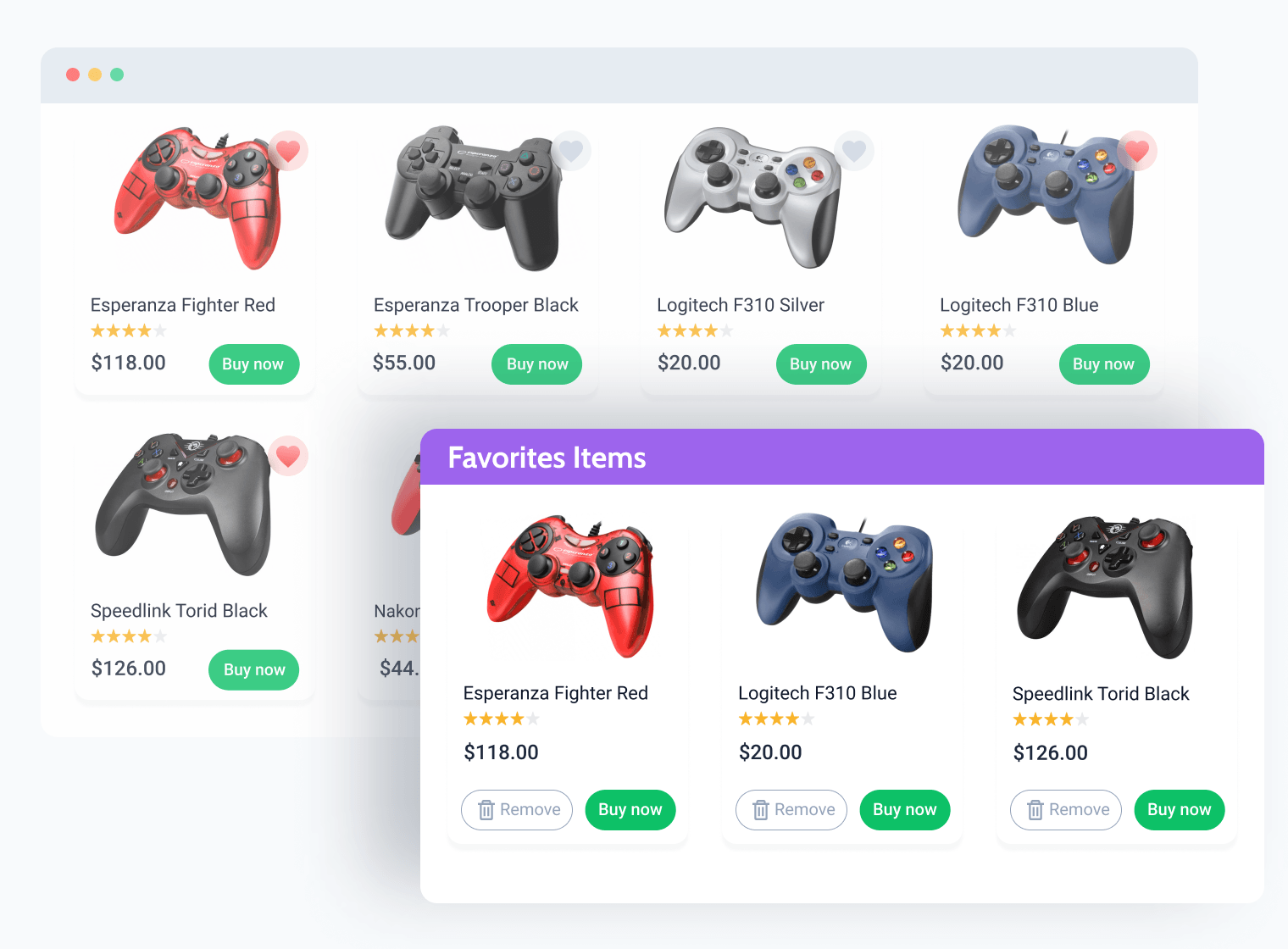The screen displays an online shopping interface for handheld game consoles and accessories. In the background, there's a grid listing various gaming items. A prominent pop-up banner labeled "Favorite Items" in white text on a purple strip is visible on the left side. This banner features three game controllers: one red, one blue, and one black.

1. **Red Controller**:
   - **Name**: Esperanza Fighter Red
   - **Rating**: 4 stars
   - **Price**: $118
   - **Buttons**: "Remove" (white with gray text and outline) and "Buy Now" (green with white text)

2. **Blue Controller**:
   - **Name**: Log Tech F310 Blue
   - **Rating**: 4 stars
   - **Price**: $20
   - **Buttons**: "Remove" and "Buy Now"

3. **Black Controller**:
   - **Name**: Speedlink Taurid Black
   - **Rating**: 4 stars
   - **Price**: $126
   - **Buttons**: "Remove" and "Buy Now"

Beneath the pop-up, the main list features more items arranged in a two-row grid. Only the top row and part of the bottom row are visible. The top row includes:
   - **Esperanza Fighter Red**: $118 (same as in the favorite items)
   - **Esperanza Trooper Black**: 4 stars, $55
   - **Log Tech F310 Silver**: 4 stars, $20
   - **Log Tech F310 Blue**: $20

These items only have "Buy Now" buttons without the "Remove" option.